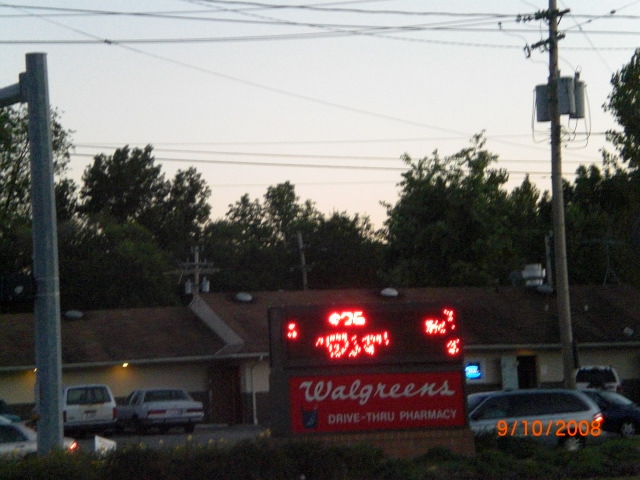The image prominently features a Walgreens sign in the foreground at the bottom center. The sign is a vivid red with the word "Walgreens" displayed in their signature cursive white font. Beneath this, the text "drive-thru pharmacy" is written, and to the left of this text is a dark icon resembling a pharmacy jar or container filled with liquid, symbolizing pharmaceutical services.

Surrounding the sign, various cars are visible. One car, a small gold-colored vehicle, appears to be in operation as indicated by its illuminated red taillights. The exact color of the car is somewhat obscured by the lighting, giving a potentially different hue. Just behind the sign, a gray minivan and another car can be seen partially peeking out.

In the background, several vehicles are parked in front of a long building. This building is beige with a dark brown roof and serves as the backdrop to the sign. Trees with dark leaves frame the scene, with an evening or twilight sky casting a serene atmosphere over the image.